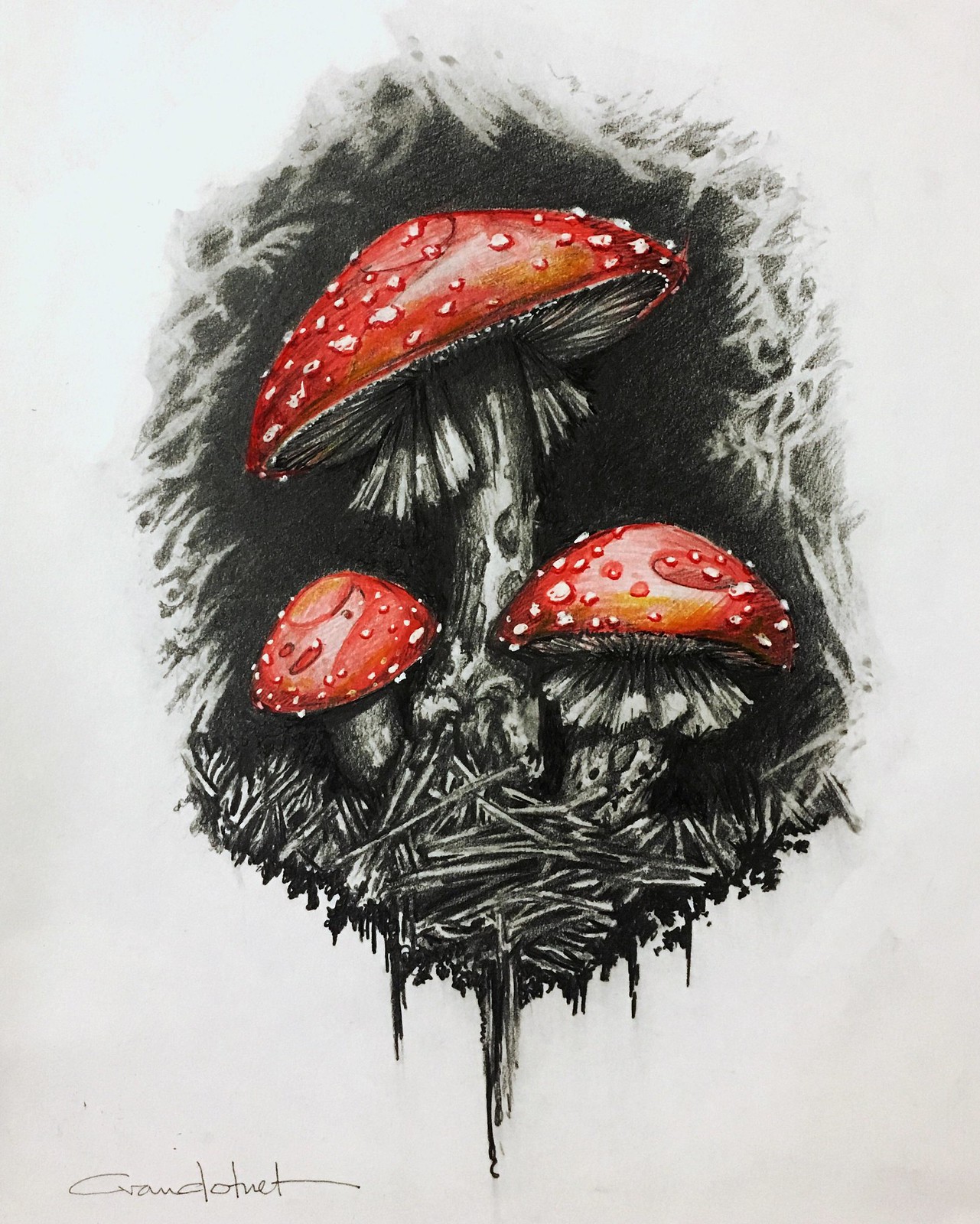This image, which could be mistaken for a tattoo, showcases a detailed drawing on a light gray background. It features a black cave-like cutaway filled with delicate white foliage and an assortment of black twigs and sticks, providing a dark, forest floor contrast. Centrally framed against this backdrop are three mushrooms of varying sizes, each with gray stems and striking red caps adorned with white dots. The caps display moisture droplets, suggesting recent rain or dew. The smallest mushroom rests on the left, accompanied by a stem that bridges to the slightly larger mushroom on the right. Dominating the composition is the tallest and largest mushroom, positioned high at the center. The piece is signed in black pencil or pen on the left side.